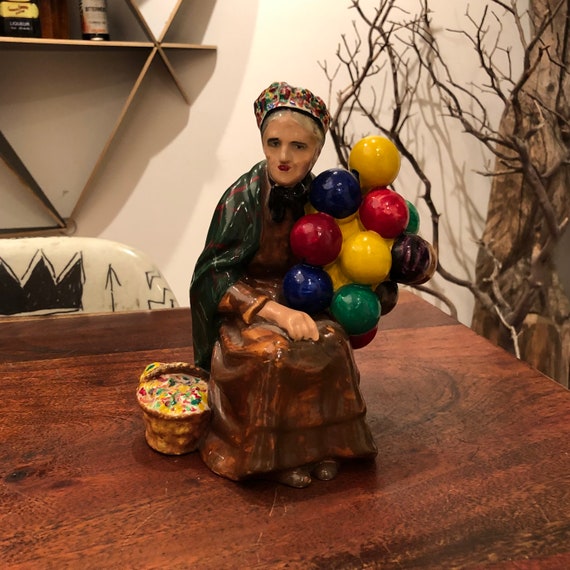In the foreground of the image, there is a meticulously sculpted figurine of an elderly woman seated on a finely polished, dark brown wooden table. The woman is depicted wearing a long brown dress with a black tie at the neck, a colorful cap with hues of white, green, red, yellow, and blue, and a green jacket draped over her shoulders. She holds a vivid array of balloons in her arms, consisting of yellow, red, blue, green, purple, brown, and some obscured by her figure. At her side is a brown basket, filled with assorted colorful items.

The background showcases a white wall adorned with a triangular wooden shelf positioned in the top left corner. The shelf holds a black bottle with a white label, and to its left, two boxes—one yellow and black. Below the shelf is a white chair that features a black crown and arrow design, indicating detail in black text that is not fully legible. To the right side of the image, there is a display of cured branches arranged as a decorative bare tree.

Overall, the scene exudes the charm of a collector's item or museum piece meticulously set in a homely yet artful arrangement.